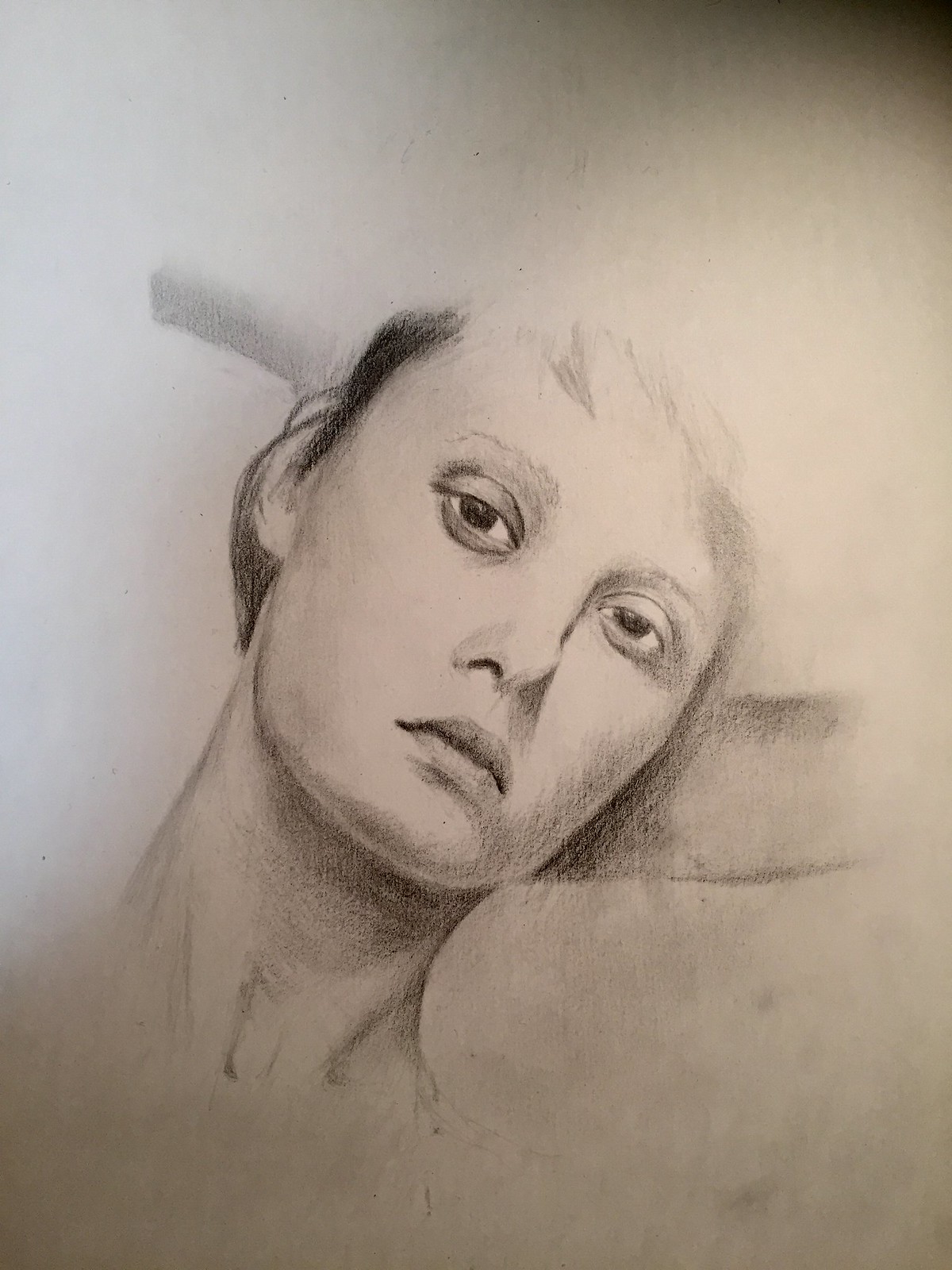The image appears to be a highly detailed pencil drawing on a grayish background. At the center, it features a portrait of a woman with her head tilted slightly to the right. Her hair partially covers her forehead with bangs and flows over her ears on the sides. Her dark, heavy-lidded eyes exude a deep sense of emotion. She is depicted with full lips and pronounced shading on the right side of her face and neck, adding a sense of depth and realism to the image. Although it seems like she might have an arm extended behind her, the focus remains on her head and neck. The shading along her neck accentuates strong, well-defined muscles, contributing to the intricacy and lifelike quality of the drawing.